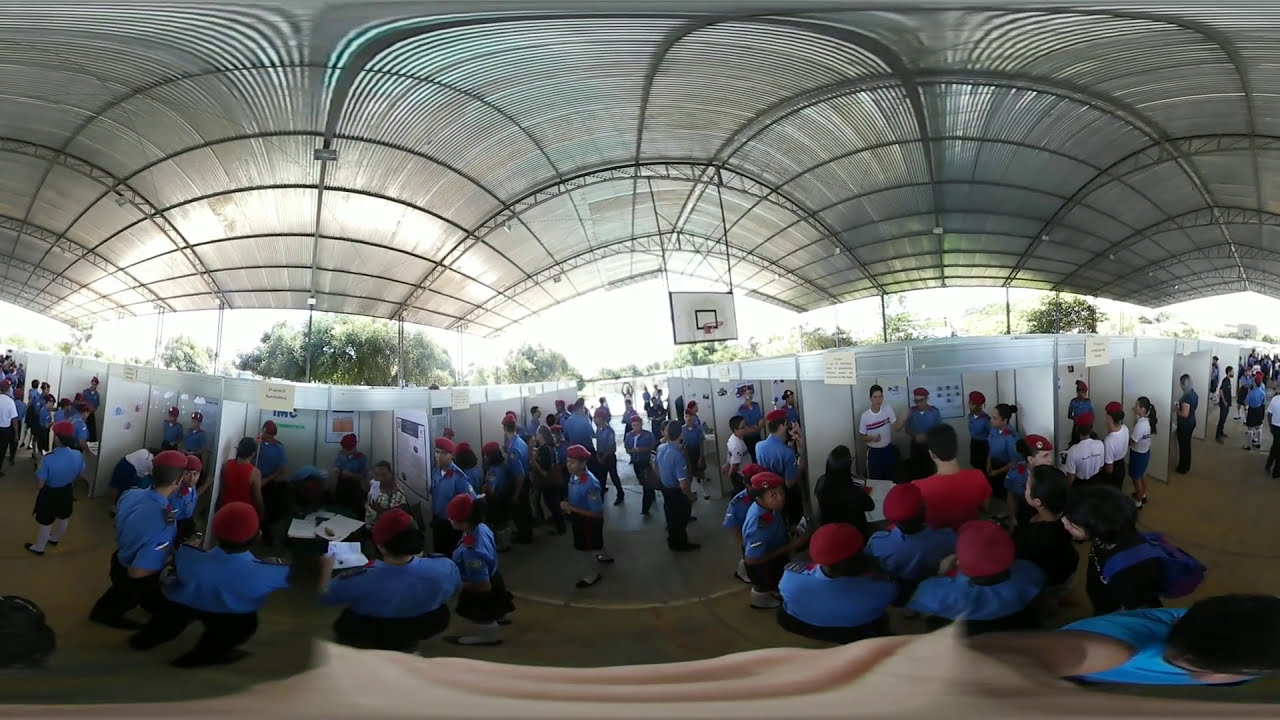This photograph captures a bustling event within a large, gymnasium-like space, possibly set up for a job fair or similar gathering. The high-arched ceiling, supported by metal structures, suspends basketball hoops with white backboards, signifying the gymnasium's typical use. The venue is intricately arranged with numerous white partitioned sections or booths, extending both laterally and deeper into the background, each evidently designated for different recruiters or exhibitors.

The majority of the attendees appear to be uniformed, wearing blue short-sleeve button-down shirts, black or dark pants, and distinctive yellow caps. Another group of uniformed individuals can be seen in light blue shirts and red berets, which could imply an affiliation with a military school or a similar institution. Interspersed among these uniformed participants are a few attendees in civilian attire, as well as some people in white t-shirts, contributing to the diverse fabric of the event.

The tented roof of the venue, looping and curving overhead, partially shelters the interior but reveals glimpses of the bright, blindingly white sky outside through openings, enhancing the natural light within. Despite the brightness outside, the indoor lighting creates a somewhat dim, dark-beige ambiance on the floor, obscuring finer details. The space is animated with movement as attendees navigate through the booths and partitions, engaging with various stands and displays, emphasizing the active and interactive nature of the event.